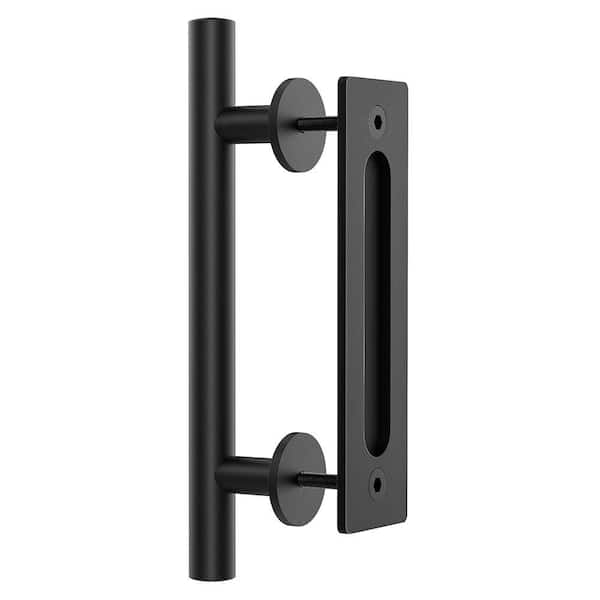In the image, a sturdy metal bracket is showcased against a pure white background. The bracket is predominantly black and appears to be quite heavy. From the left side, a thin black vertical bar rises, connecting to several smaller horizontal bars that feature circular discs. These discs, positioned near the top and bottom of the bracket, have small black pegs extending from them. These pegs secure a single, vertically elongated rectangular panel on the right side. This black rectangular piece is long and narrow with a hole at both its top and bottom, possibly for screws, and features a hollowed-out, pill-shaped cutout in its center. The cylindrical grip handle part, connected through the circular discs, suggests it could function as a robust door handle.